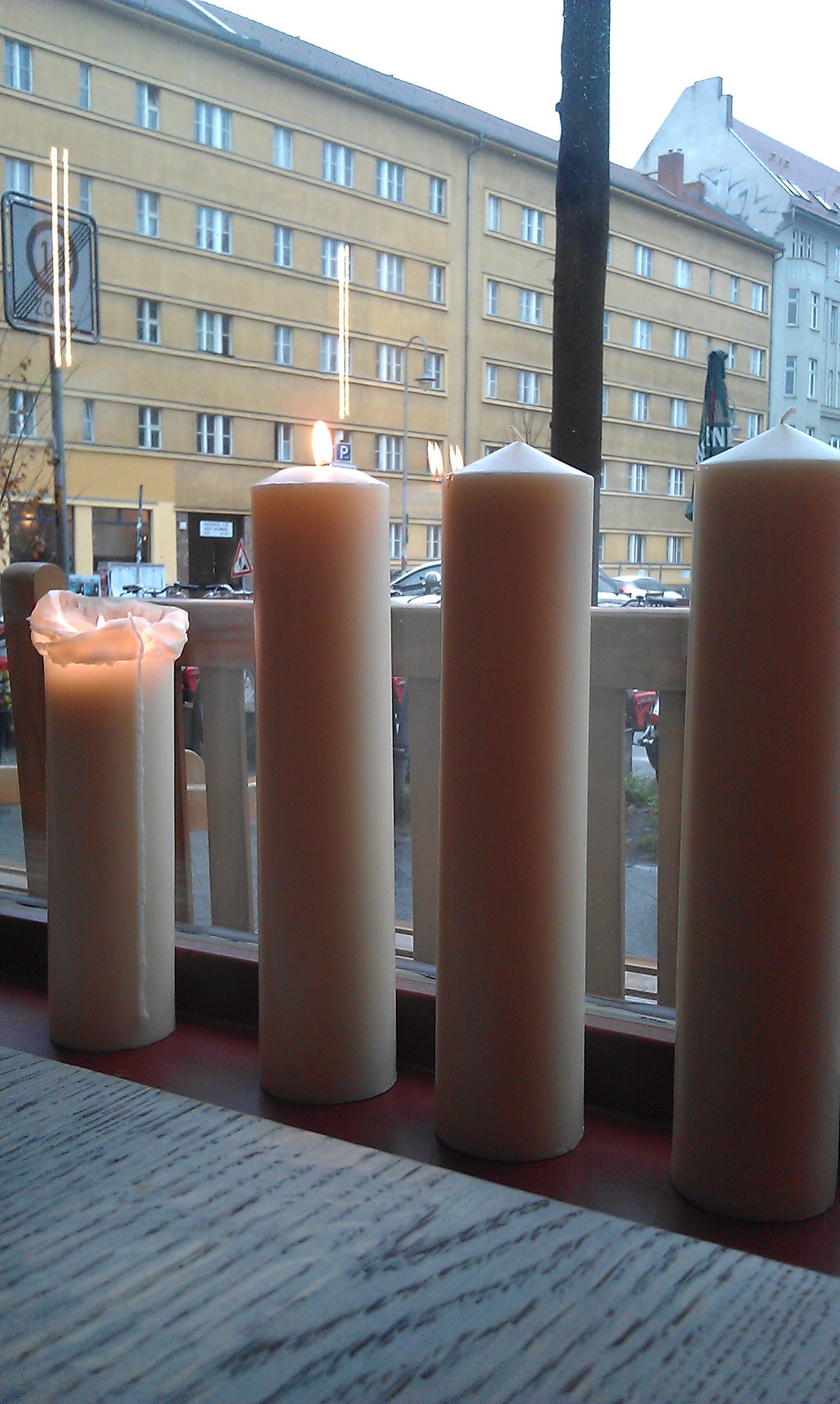This detailed image features four large, cylindrical wax candles arranged on a windowsill against an expansive window. Each candle is tan in color and varies in its state of use. The candle on the far left is the shortest, with wax heavily melted down about a third of the way and currently lit, with wax visibly dripping. The second candle from the left is also lit, appearing freshly ignited. The two candles to the right remain unlit and untouched. Beneath the candles, the surface appears to be a reddish, wooden ledge or table. The foreground reveals a carpet with an off-white and black striped pattern, resembling a zebra print. Through the window, the cityscape includes multi-storied apartment buildings. One prominent structure has a yellowish facade with numerous small windows and is perhaps five to six stories tall. Adjacent to it on the right is a slightly taller building with a light blue exterior. Further details, such as street signs and what might be a Guinness flag from a restaurant patio, are visible, indicating a busy street below. The sky appears overcast, contributing to the scene's ambiance.